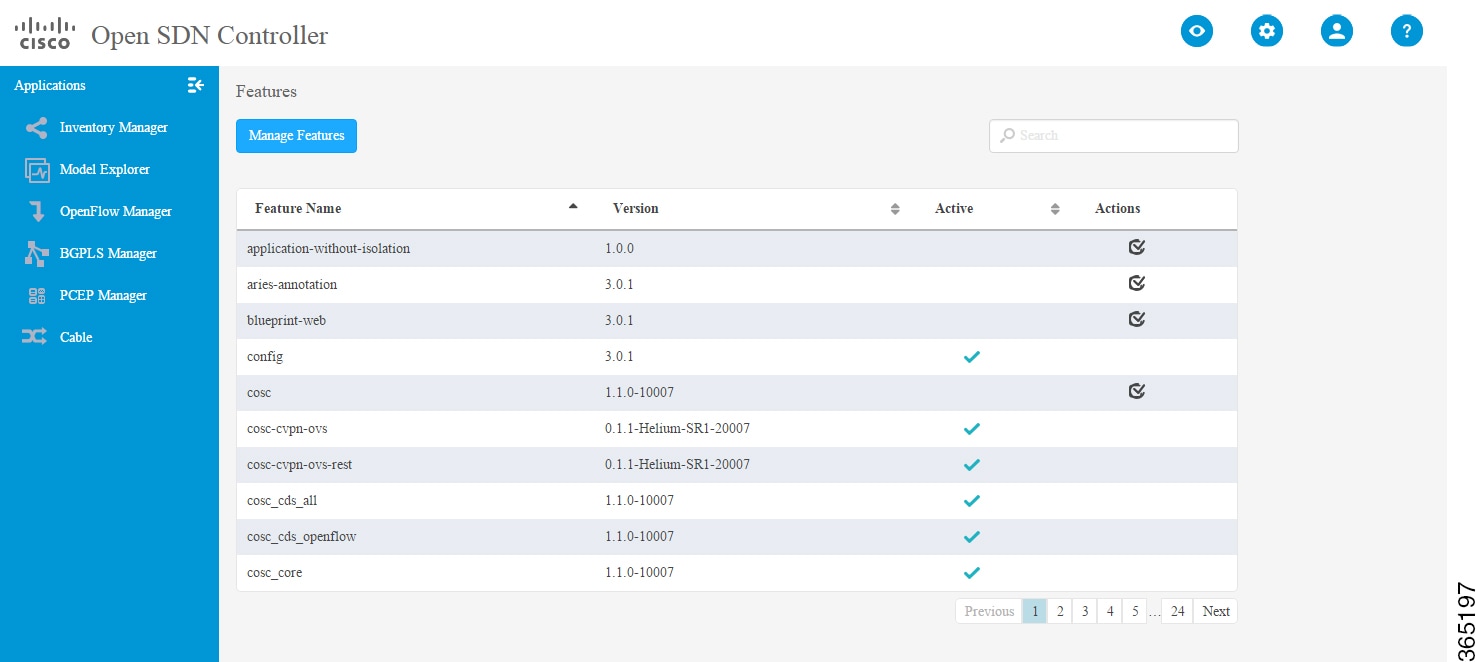In this screenshot, set against a white, light gray, and blue background, the upper left corner prominently features the Cisco OpenSDN controller. Beneath this label, a blue vertical box displays light blue text reading from top to bottom, listing various components: Applications, Inventory Manager, Model Explorer, OpenFlow Manager, BGPLS Manager, PCEP Manager, and Cable.

To the right of this vertical list, at the top, there is a section labeled "Features." Directly below this label, another blue box contains the text "Manage Features." This section is organized into columns from left to right, labeled: Feature Name, Version, Active, and Actions. 

An example from this list includes the first line item: "Application Without Isolation" with Version 1.0.0. Following entries include "ARIES Annotation" with Version 3.0.1, and "Blueprint Web" with Version 3.0.1.